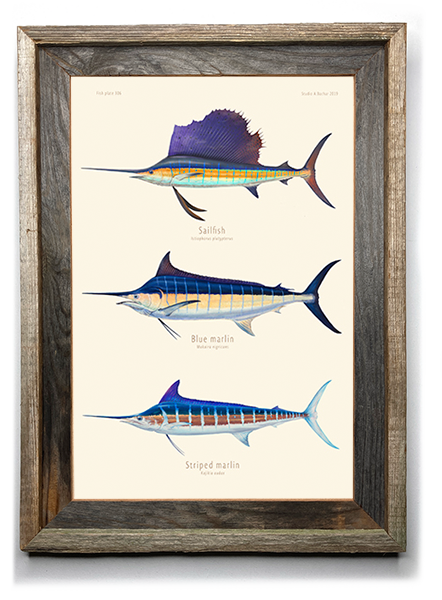The image is a framed piece of printed art, housed within a worn light brown wooden frame. Inside the frame is a brown mat bordering the artwork. The print, set against an off-white background, features three saltwater fish arranged vertically. At the top is a sailfish, distinguished by its huge fin and a blend of dark blue, purple, light blue, and orange colors. The middle position is occupied by a blue marlin, which showcases dark blue stripes, shades of blue, whitish gray, and touches of light orange. The bottom fish is a striped marlin, noted for its lighter blue hue, brown base, and a smaller sword-like snout. Each fish is depicted in realistic, vibrant colors, accurately representing the natural appearance of these species.